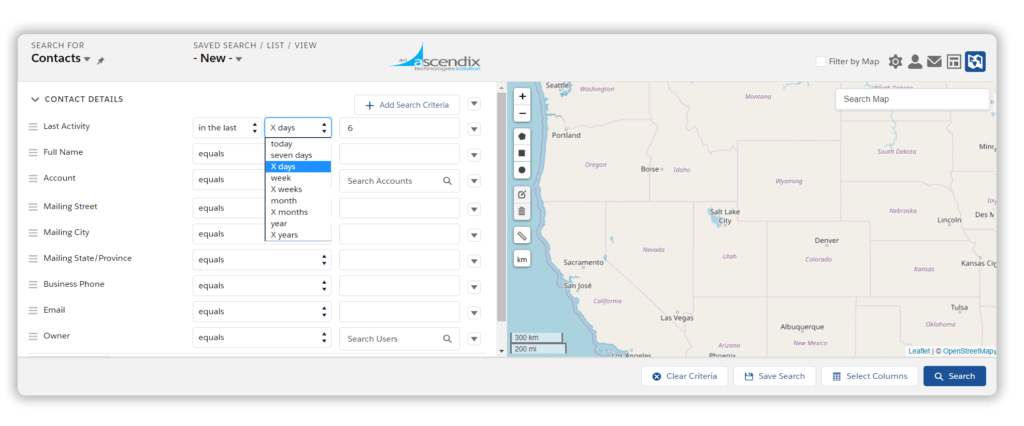A detailed screenshot from the ASCENDIX platform showcases the Contacts menu. The interface is divided into two distinct sections: the left part displays contact details, while the right part features a map. The sections are aligned side-by-side, meeting at the center. At the top left, a search bar labeled "search for" is visible, with "contacts" displayed below. Adjacent to this, there's a sizable area labeled "Save to search/list/view," followed by a button labeled "new" with a dropdown arrow. The map on the right prominently displays Salt Lake City at its center.